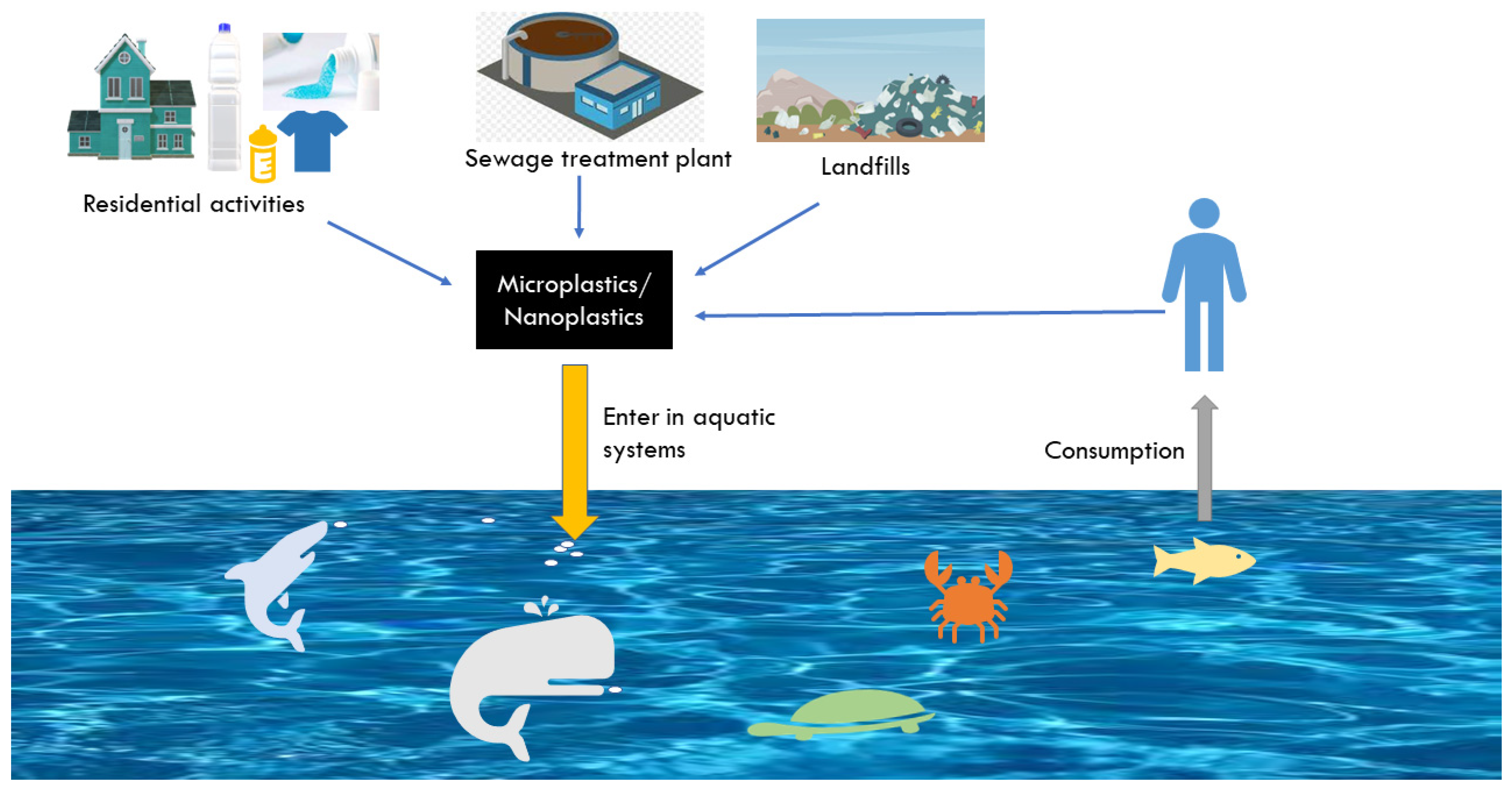This detailed scientific infographic, reminiscent of textbook diagrams, illustrates the journey of microplastics and their impact on ocean ecosystems. The top-left corner features a residential area depicted by a blue two-story house surrounded by household items like a t-shirt and water dispenser, captioned "residential activities." To the right, an image of a sewage treatment plant labeled "sewage treatment plant" shows another source of microplastics. Further right, a landfill with mounds of garbage is captioned "landfills." Blue arrows from these three sources converge on a central black box labeled "microplastics/nanoplastics," indicating their origin. A yellow arrow beneath this box points downward, labeled "enter in aquatic systems," showing how these particles enter marine environments. In the ocean section at the bottom, clip art images of marine wildlife, including a white whale, blue shark, green turtle, orange crab, and yellow fish, demonstrate the affected sea life. Above the yellow fish, a gray arrow points toward a blue stick-figure human icon, with another arrow leading back to the central box, labeled "consumption," highlighting the circular journey of microplastics from human use back to human consumption through aquatic food chains.